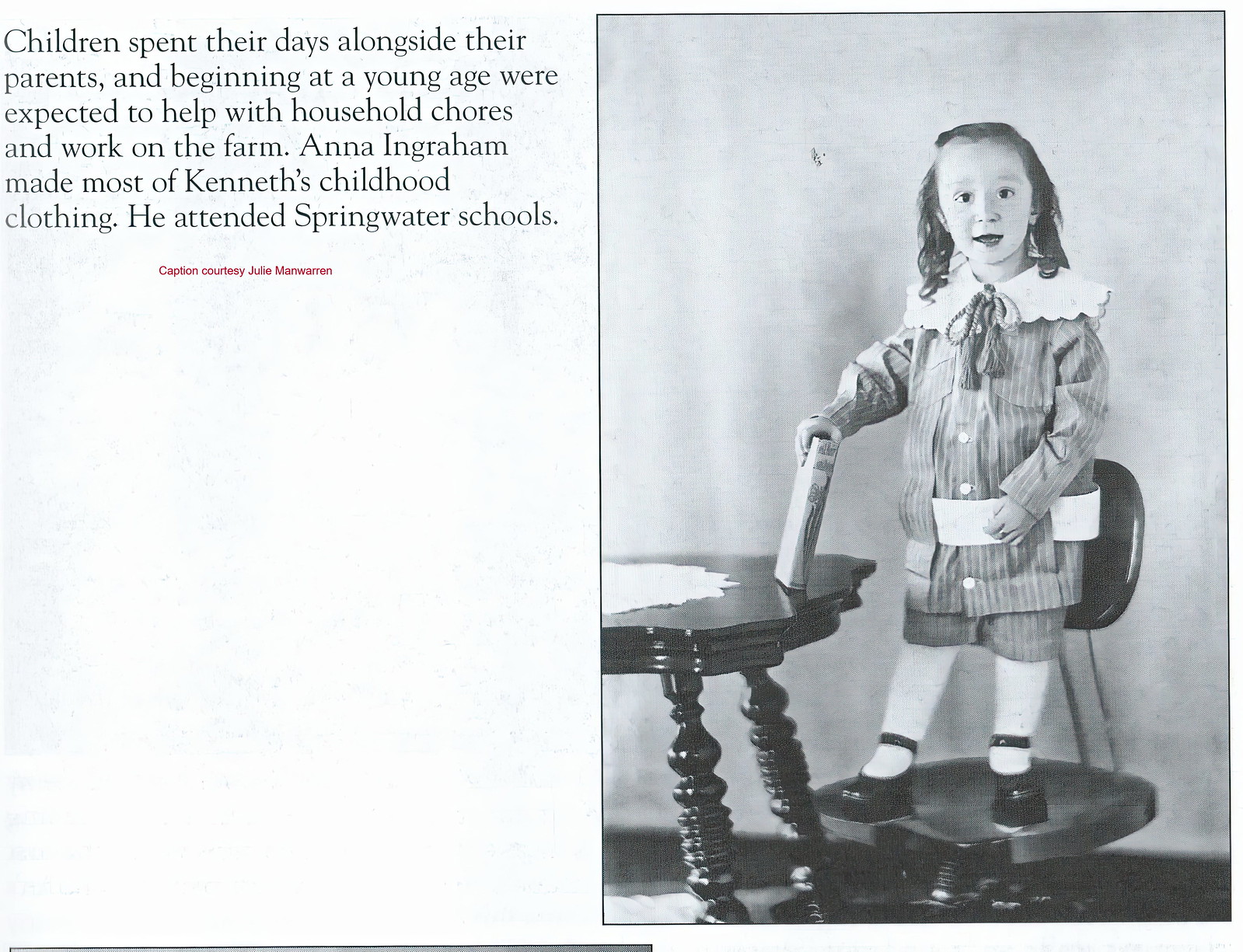In this black-and-white photograph, taken from a book in landscape orientation, the right half features a meticulously detailed vintage portrait of a young child. The child, approximately four years old, is standing on a chair and holding a book in their right hand, which is resting on an ornately carved wooden table adorned with a doily. The child has longer, curly hair and is dressed in an antique sailor-type suit with stripes, slightly oversized shorts, white tights, and black shoes resembling Mary Janes. The outfit is completed with a large scalloped collar and a corded closure. The left half of the image contains text on a light gray background, describing the context of the photograph. The black text reads: "Children spent their days alongside their parents and beginning at a young age were expected to help with household chores and work on the farm. Anna Ingraham made most of Kenneth's childhood clothing. He attended Springwater schools." Below this, in small red letters, is the credit: "Caption courtesy Julie Manwarren." The overall presentation exudes the style of a vintage print publication, reflecting a bygone era.